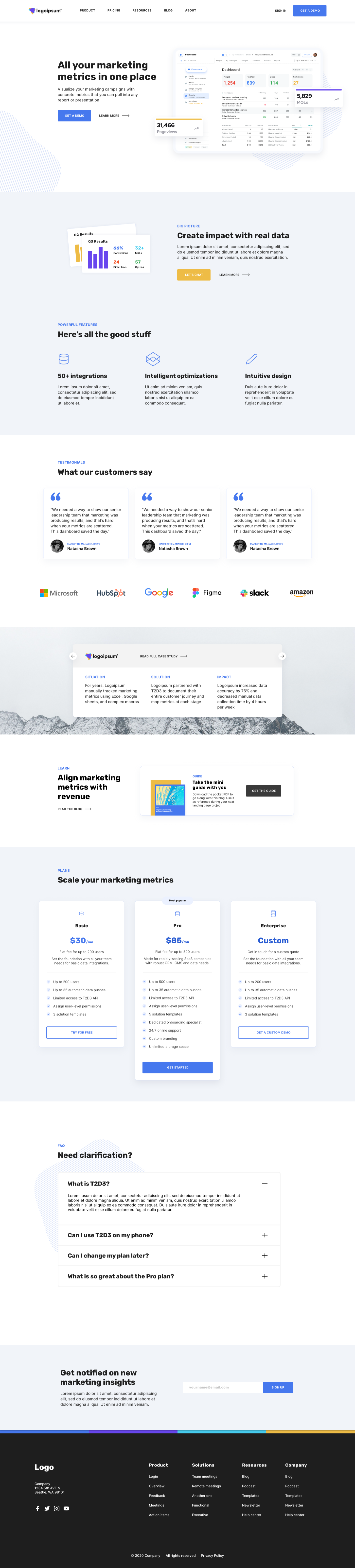The image appears to be a distorted view of a webpage, potentially showcasing elements from either a singular page or two merged pages. Although the text is difficult to decipher due to the distortion, some key elements can still be identified. 

In the upper-left corner, there is a logo reading "Logo IPSUM," accompanied by a navigation bar at the top with the following options: Product, Pricing, Resources, Blog, About, Sign In, and Get a Demo. 

Just below, a prominent section bears the headline, "All your marketing metrics in one place." It promotes the ability to visualize marketing campaigns with concrete metrics that can be included in reports or presentations. This section features a blue "Get a Demo" button and a "Learn More" link. It also mentions metrics like "31,466 page views" and "1,254" units of some undefined measure, though the precise details are unclear.

Further, the webpage highlights "50+ integrations" and contains placeholder text like "lorem ipsum," which is typically used as dummy text in design mockups. Other phrases such as "Conductor," "a disciplined elite," and "Intelligent Optimizations" are scattered throughout, although their context remains ambiguous. Despite the overall distorted and jumbled appearance, elements pointing to marketing analytics and user engagement are evident.